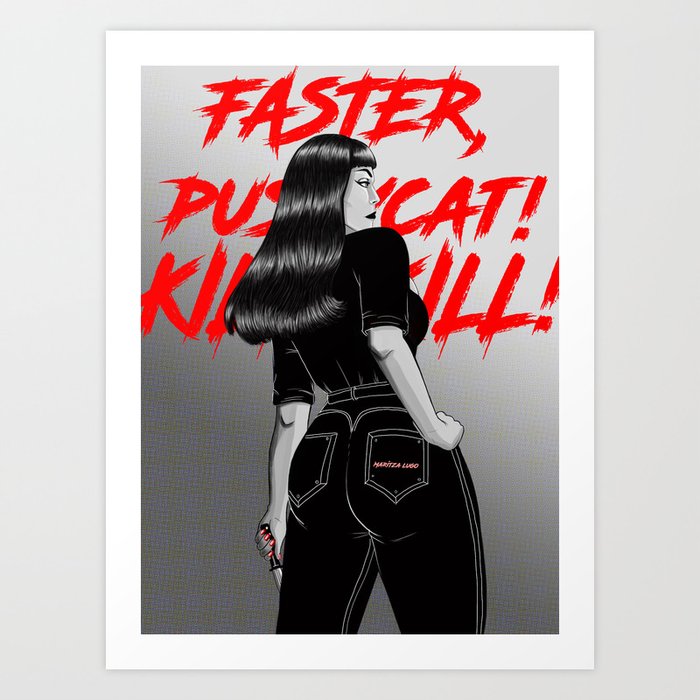The image is a rectangular poster with a white border and a gray background, featuring an artwork in the center. The artwork depicts a black and white woman with long, sleek black hair, flowing past her shoulders, and prominent eyebrows. She's wearing a black, short-sleeved shirt and black jeans with white stitching and pockets, with the name "Maritza Lugo" written in pink on the back of the jeans. She stands with her right hand on her hip and holds a knife with a black handle in her left hand, which hangs down by her side. The woman has grayish skin and closed mouth. At the top of the poster, in horror-style red paint-stroke lettering, it says "FASTER" on the first line, "PUSSYCAT" on the second line, and "KILL KILL" on the third line.